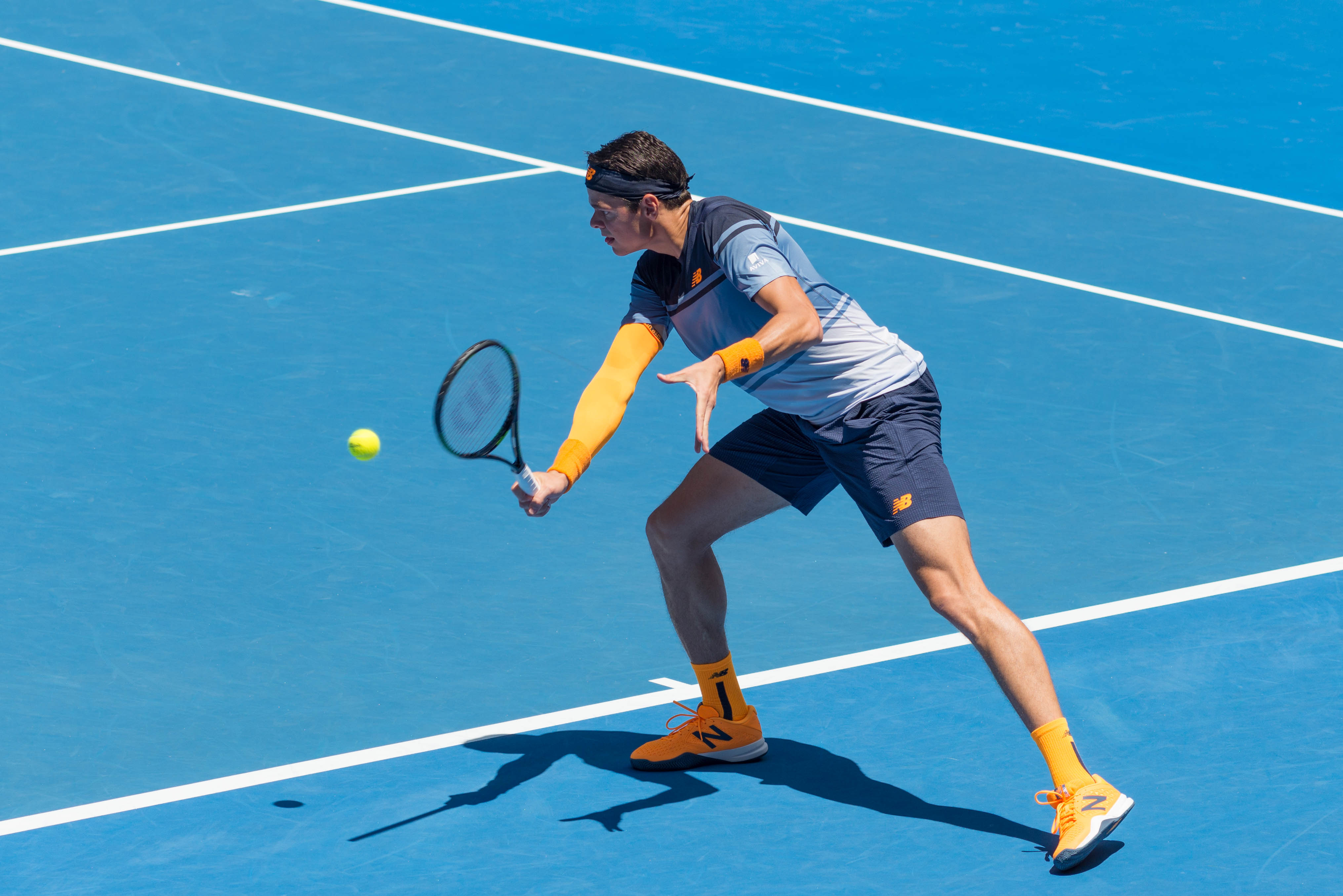In this vibrant photograph set on a sunny day, a tall Caucasian man with brown hair is intensely focused as he prepares to strike a yellow-green tennis ball on a blue and white-lined tennis court. The athlete, donning a dark blue New Balance headband, is mid-swing, stretching onto his left leg while channeling all his weight onto his right leg. He grips a Wilson racket, marked with a "W" in the center, in his right hand, covered by a yellow sleeve. His attire consists of a blue and white striped New Balance shirt, complemented by blue New Balance shorts, and orangeish-yellow New Balance shoes and socks. His shadow is prominently cast beneath him, reflecting his poised and concentrated stance.